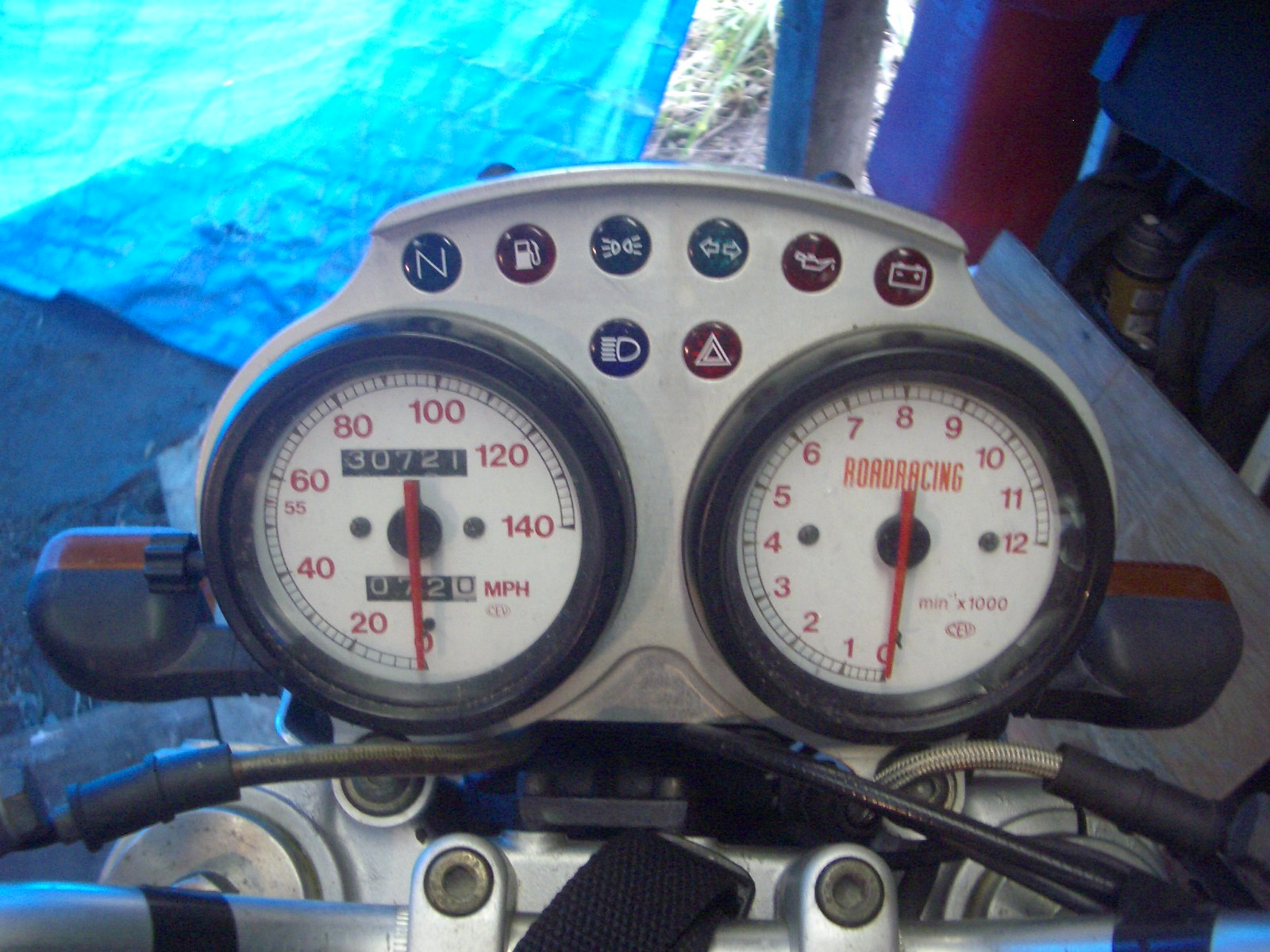The photograph captures a close-up of a motorcycle's dashboard and engine components, highlighting the intricate details of the speedometer and related indicators. The speedometer, set against a white background, features prominent red numbers and text displaying a mileage of 30,721 miles and a current speed of 72 miles per hour. Adjacent to this, another gauge, also with a white background and red lettering, pertains to road racing metrics ranging from 0 to 12, though it currently reads zero.

Surrounding the speedometer are various indicator lights for essential functions such as the neutral gear ('N'), fuel level, blinkers for both left and right turns, oil status, battery level, headlights, and an emergency alert. These indicators form a cluster across the top portion of the dashboard, none of which are illuminated at the moment. Though the intricate design of the motorcycle's handlebars is partially visible, the image focuses heavily on the dashboard, reducing the clarity of surrounding elements. The backdrop appears to be a tarp, suggesting an outdoor environment where maintenance or inspection is underway. In the periphery, signal lights on the handlebars can be detected, contributing to the overall impression of a detailed and meticulously captured scene from a stationary motorcycle.